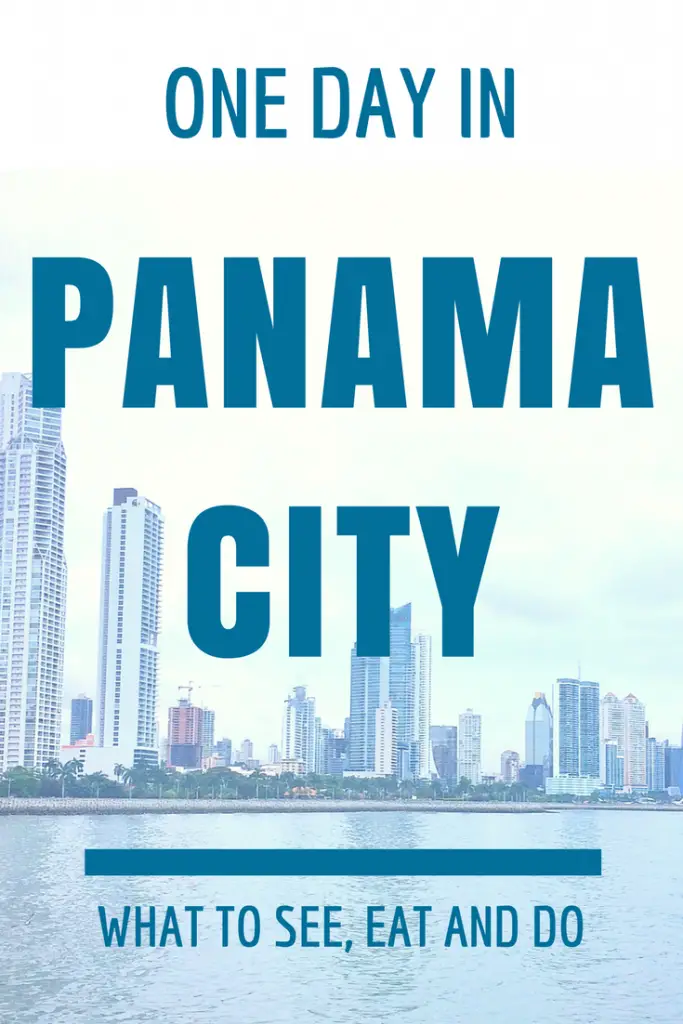The image, which is approximately 50% taller than it is wide, has the aesthetic of a poster or a well-designed website ad. The background transitions from white at the top to a very light blue about 75% down, where it sharply changes to depict water at the bottom.

In the foreground, a vibrant cityscape is displayed with an array of tall, symmetrical buildings that seem to be commercial in nature but could also be high-rise condos. These buildings rise just above the water line, occupying about 25% of the lower section of the image. The shoreline is adorned with a collection of palm trees that border a beach, leading into the water.

At the top of the image, centered in large teal letters, the text reads: "One Day In" followed by "Panama" on the next line, and "City" on the line below that. At the very bottom, a horizontal teal bar rests above the water, and within the water area, it says, "What to see, eat and do." 

The overall composition creates an inviting and informative presentation, encapsulating the essence of a day in Panama City.